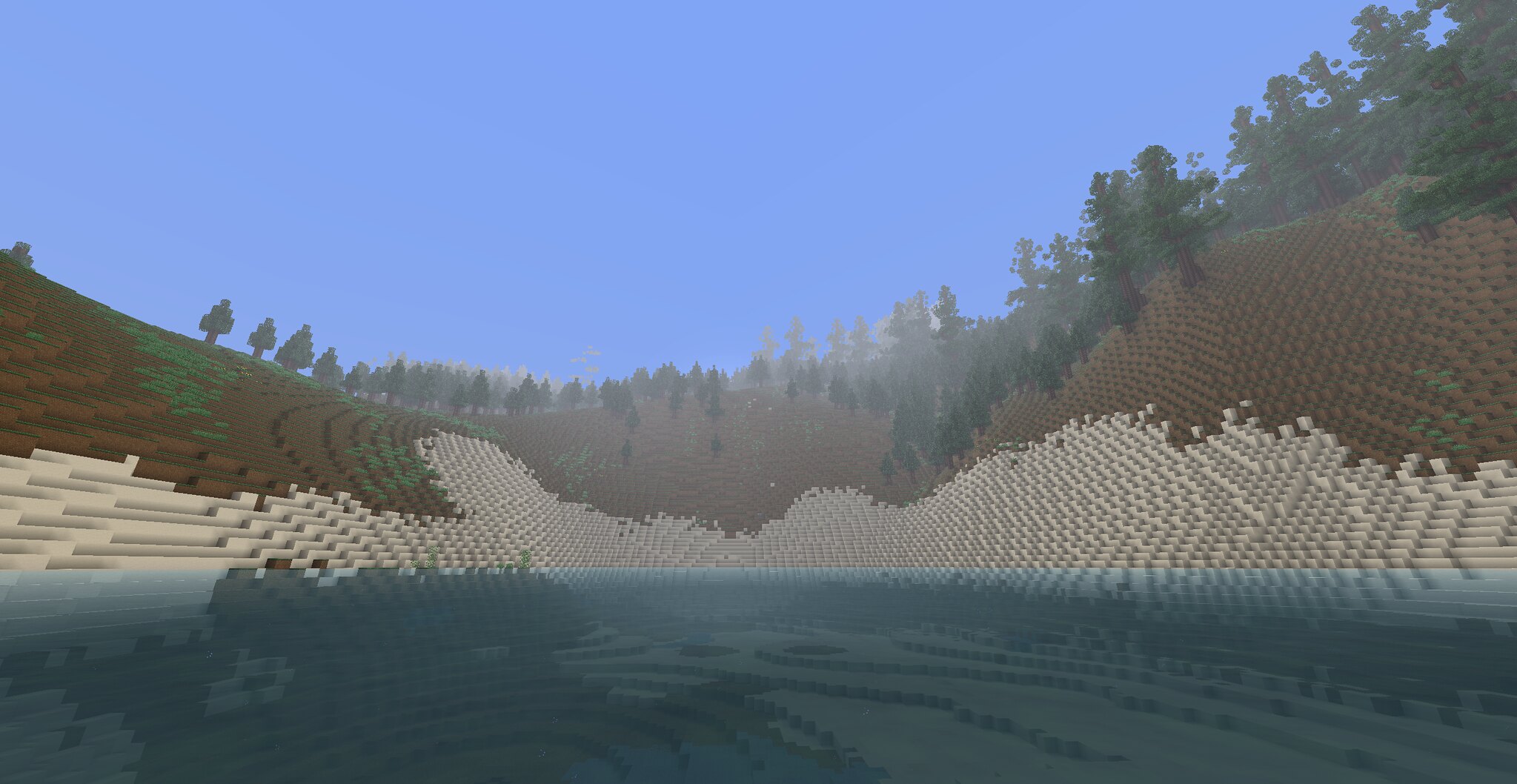The image depicts a Minecraft game screen showcasing a pixelated, blocky landscape. At the center bottom, a dark blue ocean stretches outwards, bordered by mountains and trees constructed from square blocks typical of the game's design. Along the shoreline, white sand forms staircase-like inclines towards the top right, where they meet a brown mountain adorned with more green, blocky trees. The central upper part of the image similarly features this mountainous, forested terrain. The left side of the image reveals patches of grass and soil leading to a more densely forested area, all under a bright blue sky. The entire scene, rendered in a distinctly pixelated, computer-generated style reminiscent of Lego blocks, gives off a simplistic, not very realistic, but vividly colorful appearance.